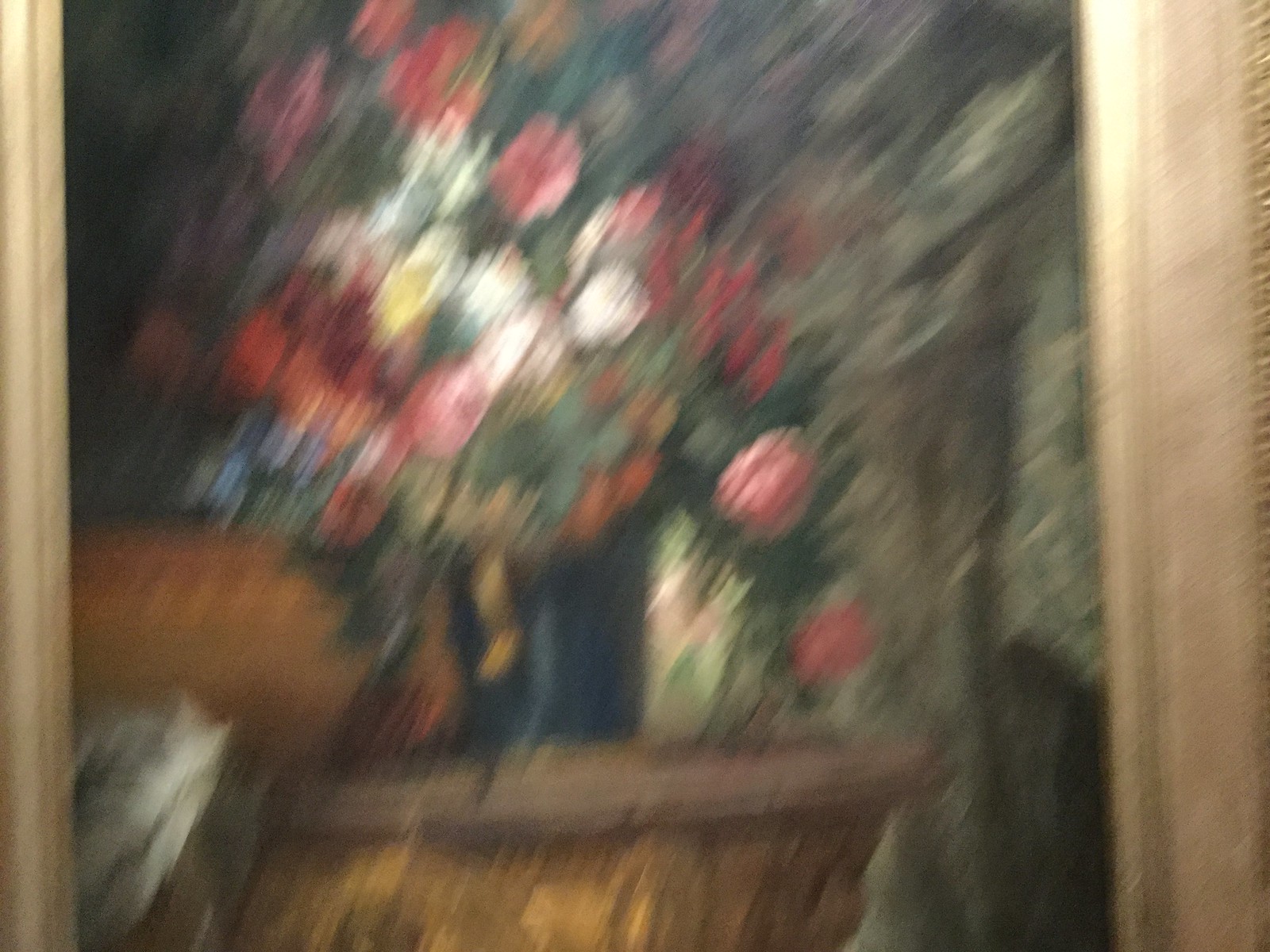This blurred image captures a partially visible painting set within a gold-colored picture frame, positioned in landscape orientation. The photo lacks a date-time stamp and appears to have been taken while the camera was in motion. Within the artwork, a basket or planter can be discerned, filled with a vibrant array of roses—yellow, red, and white—as well as hints of blue flowers. The background of the painting seems to portray a green curtain, offering a contrasting backdrop to the colorful floral arrangement, yet the overall fuzziness of the shot makes it challenging to discern specific details with clarity.